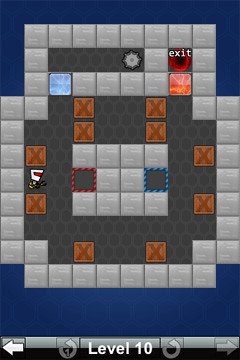This is a detailed description of a screenshot from a computer game, displayed upright in a vertical format. At the bottom of the image, "Level 10" is inscribed in white lettering, flanked by an illuminated white arrow pointing left and a dimmed arrow pointing right. Intricate swirls resembling the refresh symbol are positioned on either side of the level indicator. The background transitions from dark blue at the top to medium blue at the bottom.

The game interface consists of a grid of squares, arranged in a visually structured manner. The top and bottom rows feature eight solid gray squares each. Below the top row, the sequence is more intricate: it starts with a single gray square followed by a darker gray section containing a wheel, and then transitions to lighter gray. Among these squares, one labeled "Exit" stands out prominently.

Further details include a light blue square, a fiery square radiating orange and pink hues, and multiple gold squares marked with brown X's. A darker gray region encircles several lighter gray squares, adding to the layout’s complexity. The myriad of colors and symbols suggests varied gameplay elements within this level of the game.